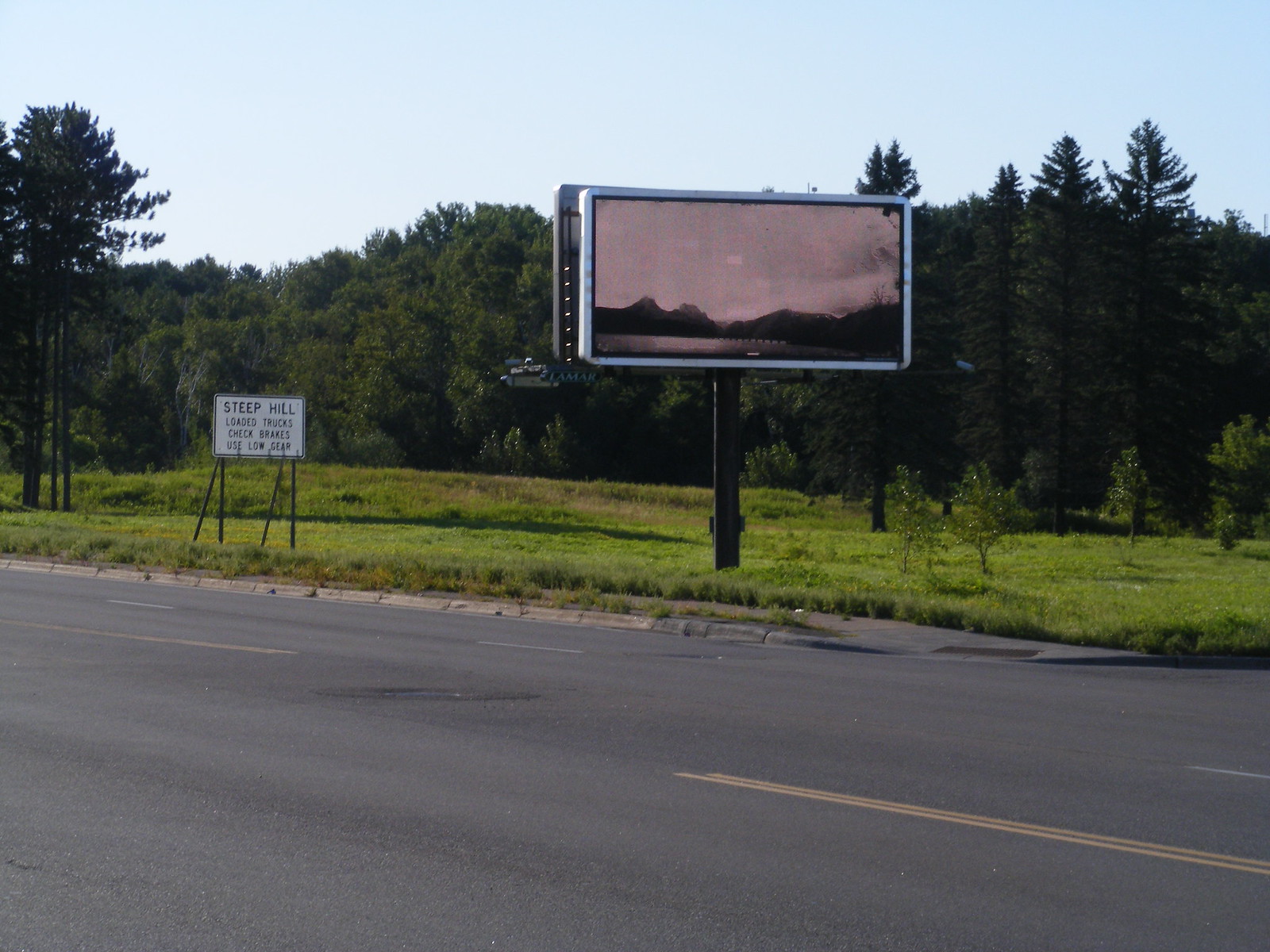The photograph captures a serene country street view. In the foreground, a multi-lane road with yellow and white painted lines stretches from the left edge to the bottom of the image. Adjacent to the street is a landscaped grassy area, recently adorned with new tree plantings. Dominating this area, a prominent billboard mounted on a wide black pole features a white frame and displays a tranquil image of a lake framed by distant hills. Ahead and to the left of the billboard, a smaller white warning sign reads, "Steep Hill - Loaded Trucks Check Brakes, Use Low Gear." The background reveals a lush line of dense foliage and towering trees under a clear, vibrant blue sky, adding to the picturesque and serene rural setting.